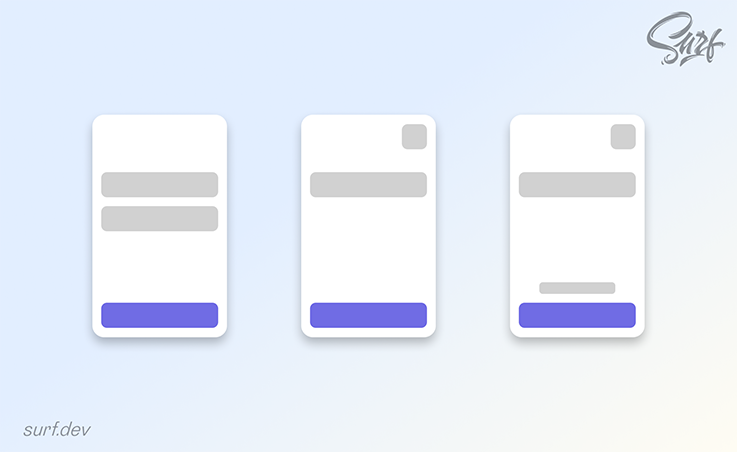The image features a soft gradient background that transitions from light blue in the top left corner to a whitish or very light blue hue in the bottom right corner. In the top right corner of the image, the word "surf" is elegantly scripted in gray cursive text. In contrast, the bottom left corner displays "surf.dev" in a legible gray font.

Centrally, the focal point consists of three evenly spaced, rectangular windows that possibly represent mobile phone screens. 

- The first window on the left showcases a minimalistic design with a white background, interrupted by two horizontal gray bars stretching through its middle, and a distinct purple bar situated at the bottom.
- The central window mirrors some elements of the first; it displays a small gray square in the top right corner, accompanied by one of the previously mentioned horizontal gray bars near the upper half, and another purple bar at the bottom.
- The third window on the right is similar but adds a small gray square positioned directly above the purple bar at the bottom, creating a subtly different layout.

The design elements collectively highlight simplicity and coherence, focused on the theme of surf.dev.